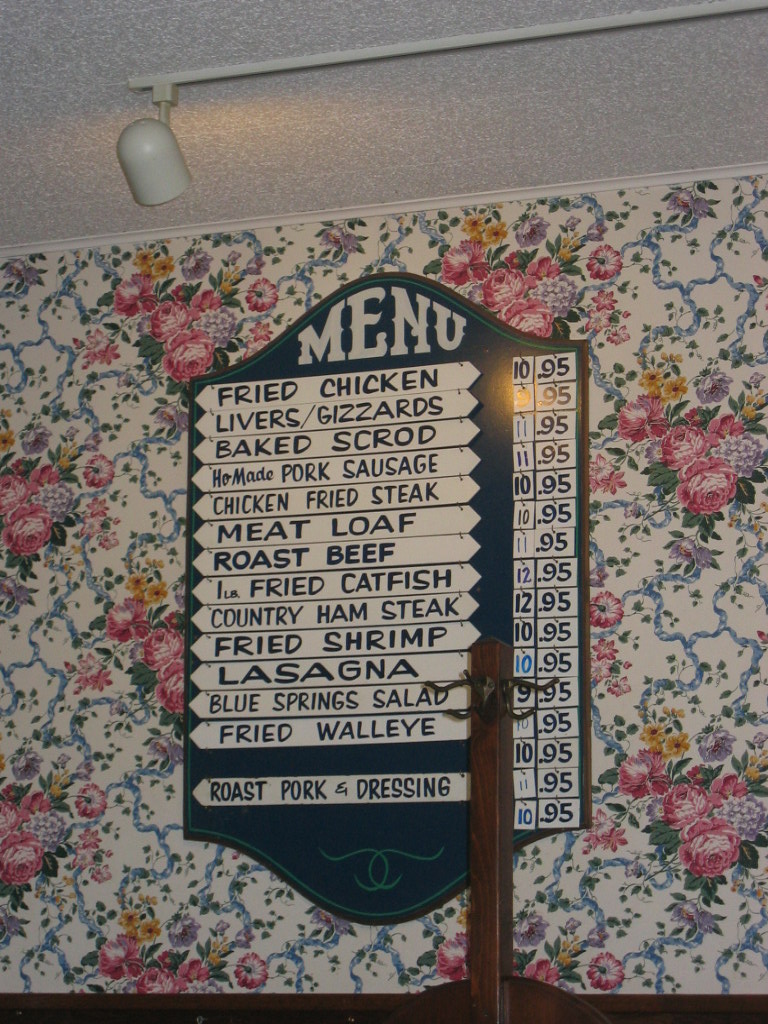This image captures a detailed restaurant menu mounted on a cast iron pole, prominently displayed against a heavily decorated, floral wallpaper. The wallpaper features a busy pattern of baskets brimming with pink roses, interwoven with purple vines that elegantly connect the floral bunches. The menu itself is affixed to a sturdy, ornate pole, with intricate metalwork serving as dividers between the sections. At the top of the menu, the word "Menu" is intricately cut out of the black metal, highlighted in white. The items are neatly listed in a vertical format with menu items aligned to the left and corresponding prices on the right. The selection ranges from "Fried Chicken" priced at $9.95 to "Roast Pork and Dressing" at $11.95. Notably, there are two additional prices listed towards the bottom without corresponding menu items, leaving a slight mystery as to what they pertain to.